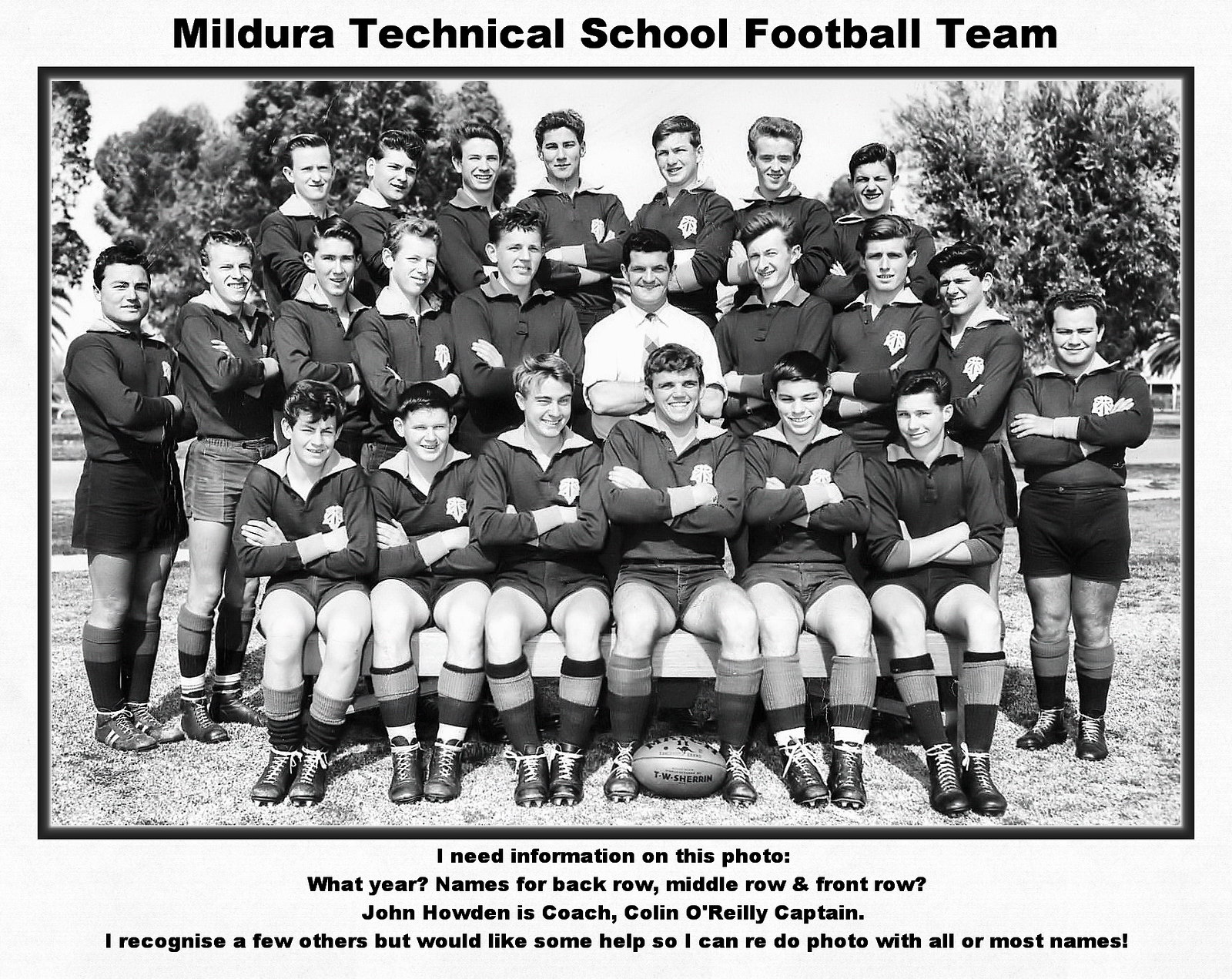This black-and-white photograph captures the Mildura Technical School Football Team, posed for a team photo outdoors on a grassy field with trees in the background. The image is framed with a thin black border nestled within a thicker light grey border. The title "Mildura Technical School Football Team" is inscribed at the top in black print. The team is arranged in three rows: the front row features boys seated on a bench with their arms crossed, the middle row of boys standing directly on the grass also with crossed arms, and the back row elevated slightly, possibly on another bench, with the same arm-crossed posture. Prominently in the middle, the coach, identified as John Howden, stands among the boys, with the captain, Colin O'Reilly, also mentioned. At the bottom of the photograph, four rows of text request further details: "I need information on this photo. What year? Names for back row, middle row, and front row? John Howden is coach, Colin O'Reilly is captain. I recognize a few others but would like some help so I can redo photo with all or most names."